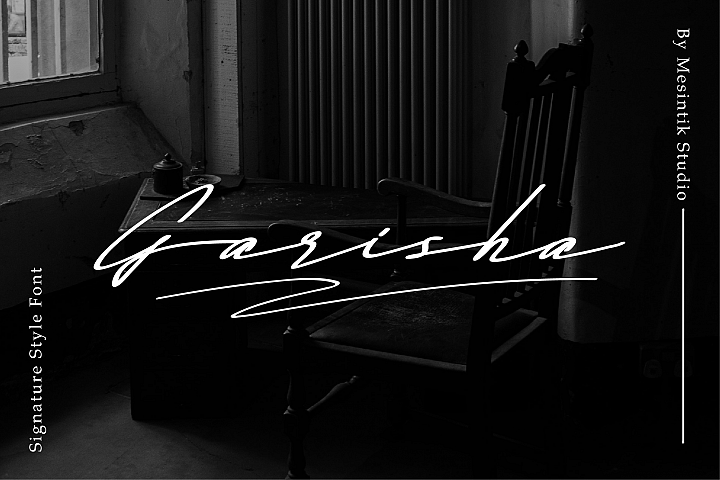The studio advertisement features a predominantly black-themed image with an old, dimly lit interior setting. On the left side, there is a vertical signature style font reading "Signature Style Font," oriented in a 90-degree angle. The most prominent text, "GERISHA," is scripted in large, white, italicized letters across the middle of the image, with a squiggle underneath. On the right-hand side, in vertical white text, it says "by MESINTIK Studio" with a line descending from the midpoint to the bottom of the image.

The image itself showcases a moody scene of a room, with a wooden rocking chair placed in front of what appears to be a weathered trunk or an old desk, both surrounded by an ambiance of neglect. A small window to the left allows minimal light to seep in, adding to the overall dark and shadowy feel. A few dishes sit atop the table, and an unusually high-mounted radiator or heater can be subtly discerned in the background, contributing to the vintage atmosphere of the room.